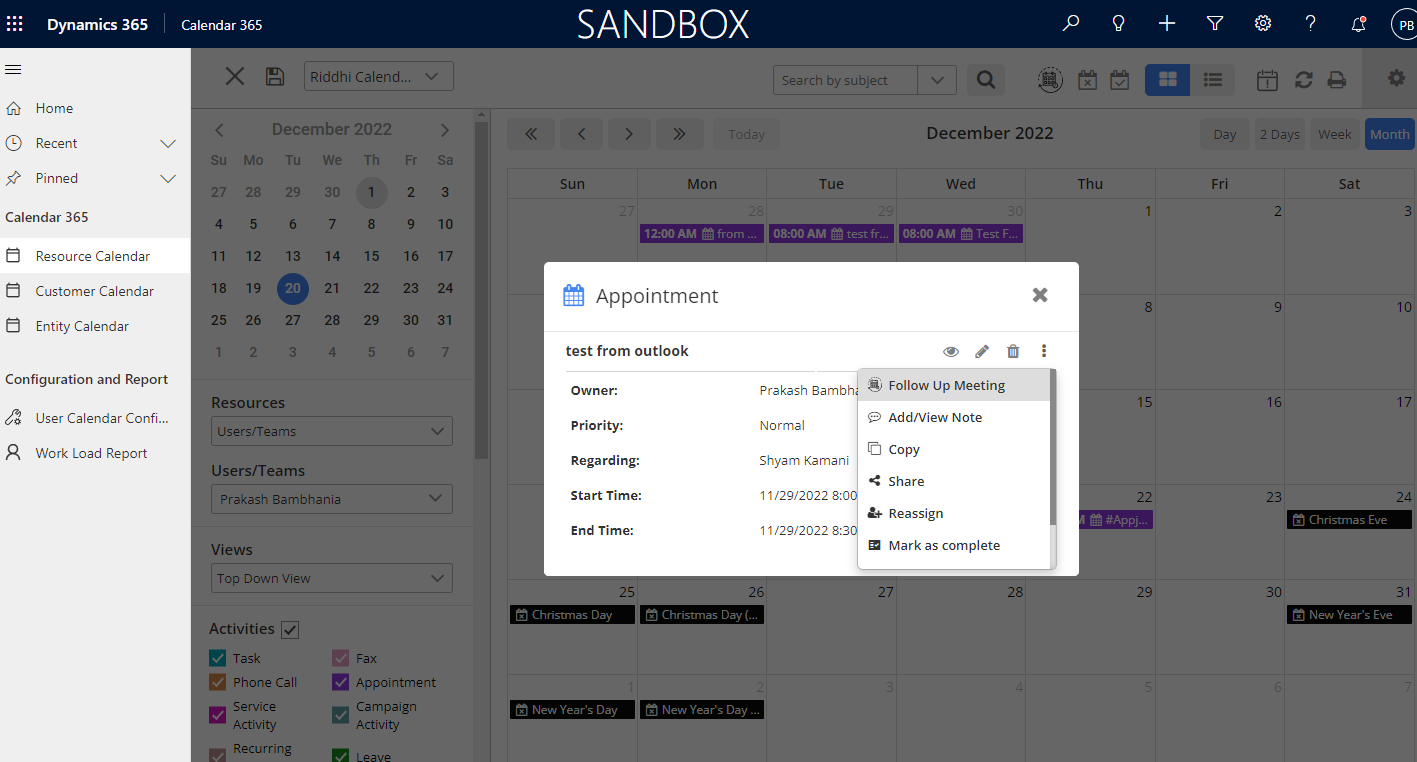The image depicts a user interface from Dynamics 365. 

On the left-hand side, there is a vertical menu set against a white background. Stretching across the top of the image from left to right is a blue bar. In the upper left-hand corner of this bar, the text "Dynamics 365" is displayed, followed by a small vertical gray separator bar. To the right of this separator, the text "Calendar 365" is visible. 

In the center of the blue bar, the word "Sandbox" is written in white font. To the right of this word, there are seven icons lined up in a row. Further to the right, the profile currently logged in is indicated by the initials "PB".

In the central portion of the image, there is a pop-up box labeled "Appointments" prominently displayed. This settings box includes several options such as the owner, priority, start time, end time, and the subject of the appointment. Users can choose to follow up, view notes, copy, share, reassign, or mark the appointment as complete from this box.